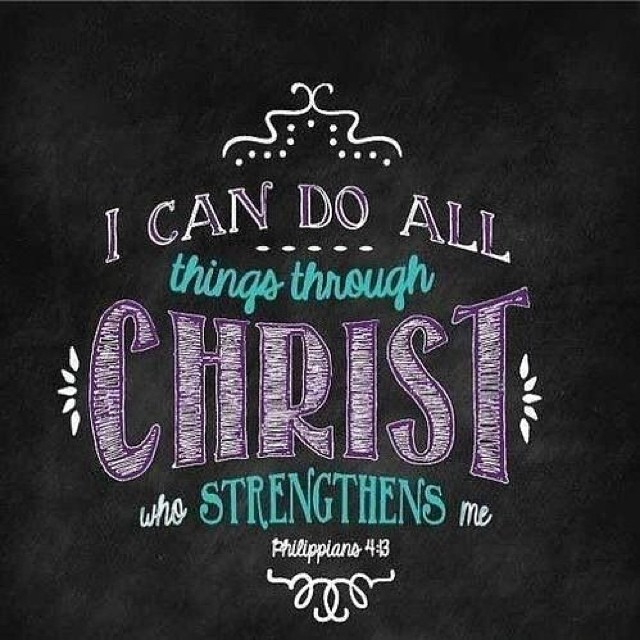This image features a striking black background with a centered Bible quote toward the bottom, positioned in the style typically found on the front of a t-shirt. The text, displayed in a mix of colors including purple, green, black, and white, reads, "I can do all things through Christ who strengthens me. Philippians 4:13." The quote is carefully arranged to cover the lower portion of the square image, standing out vividly against the dark backdrop, suggesting a design that could be used for inspirational apparel or similar items.